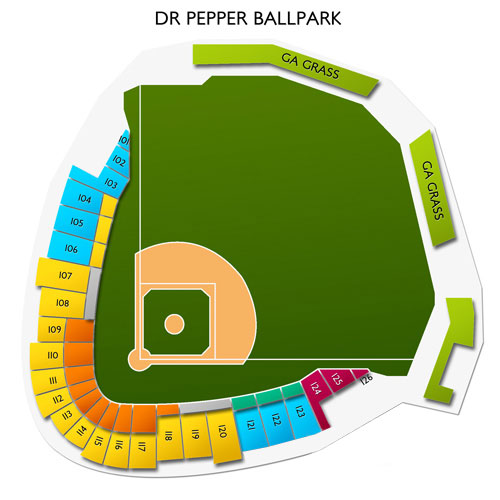The image features a detailed seating map on a white background for Dr. Pepper Ballpark. At the top, the title "Dr. Pepper Ballpark" is prominently displayed. Below the title, there is a green tab labeled "G.A. Grass." To the right of this tab, another green rectangle also reads "G.A. Grass." Below these labels, a green diagram includes a line that extends to the left before angling diagonally upward, ending with a specific end piece, likely indicating an entry or viewing point.

To the left of this diagram, the baseball field layout is shown. The field is depicted in green, representing grass, with a tan-colored pitcher's mound and additional tan areas likely symbolizing the base paths and infield. Surrounding the field are blue sections in the bleachers, labeled with seating numbers 101 through 106. Adjacent to these are gold sections numbered 107 through 120, providing a visually distinct seating area. Additional blue sections are further numbered 121 through 123. There are also purple sections, although their specific labels aren't completely detailed in the description. 

The map serves as a comprehensive guide to the seating arrangements and field layout at Dr. Pepper Ballpark, making it easy for visitors to locate their seats and general areas within the stadium.